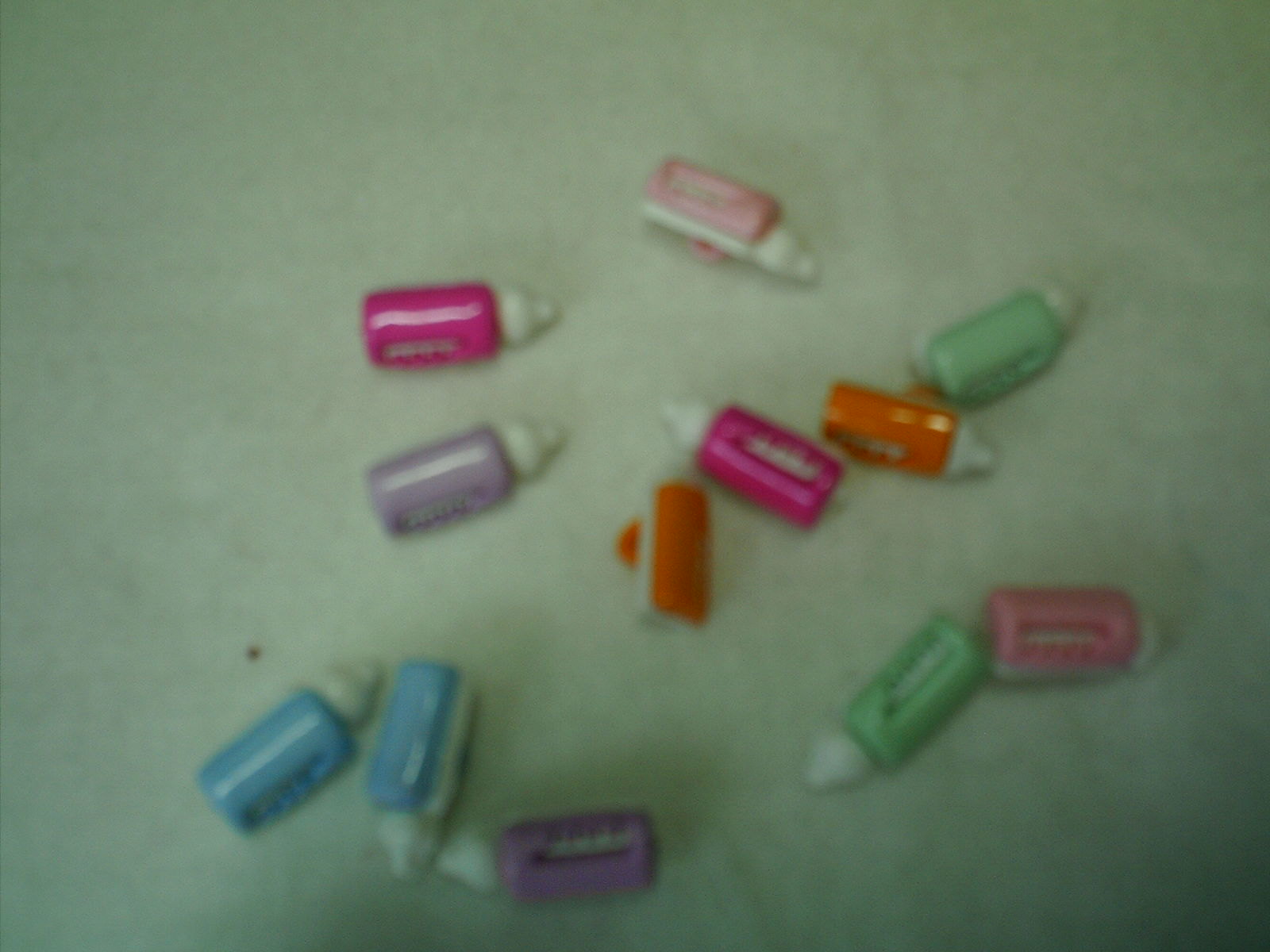This is a color photograph capturing a collection of small, miniature bottles scattered haphazardly on a table. The table has a very light greenish-gray hue. These plastic bottles, reminiscent of eye dropper or baby bottles due to their white plastic caps, come in a variety of vivid and pastel colors. The palette includes lighter pinks, darker hot pinks or magentas, very light lavender purples, burnt oranges, light pale greens, and light pale blues. The arrangement appears random, with a total of approximately ten bottles casting soft shadows on the white background, which appears darker in the bottom right corner of the image. The photograph has a slightly grainy and blurry quality, adding a subtle texture to the composition.